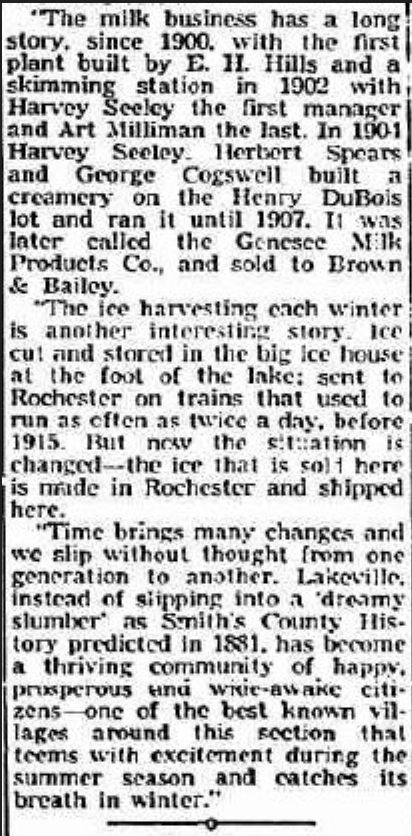The image shows a digitally scanned, rectangular newspaper clipping on a white background, bordered by a thin black line. The clipping consists of three equally-sized paragraphs of black text, although some parts of the text exhibit distortion and varying darkness, indicative of scanning imperfections. The article begins with the sentence: "The milk business has a long story since 1900," and discusses historical details such as the first plant built by E.H. Hills, a skimming station managed by Harvey Seeley in 1902, and a creamery initiated by Harvey Seeley, Herbert Spears, and George Cogswell in 1901, later becoming the Genesee Milk Products Company. The second paragraph shifts focus to the winter ice harvesting tradition, describing how ice was cut, stored in a large ice house at the lake's foot, and transported to Rochester by train, a practice that has since evolved with modern changes. The third paragraph reflects on the passage of time and community developments, noting that Lakesville has transitioned from an anticipated tranquil village to a bustling, prosperous community known for its vibrant summer activities. The text is punctuated by a horizontal line at the bottom, marking the end of the article.